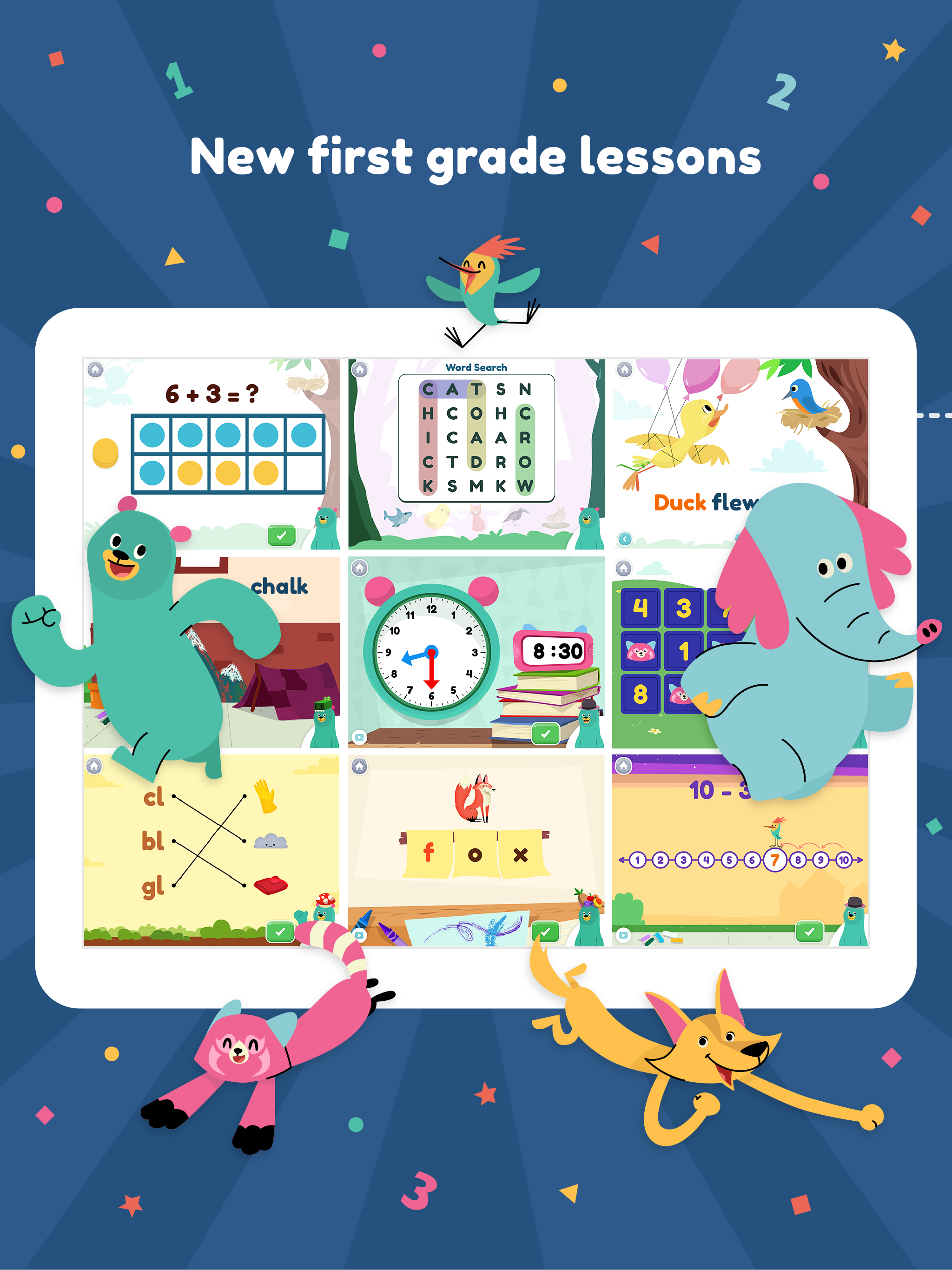This image captures a screenshot from a child's learning app designed for first graders. The background features a light blue backdrop accentuated by dark blue sun rays projecting from the center. Occupying the top central area of the screen, a bold, white text announces: "New First Grade Lessons."

Beneath this text, there is a prominent white iPad displaying nine distinct thumbnails arranged in a grid of three rows. Each thumbnail represents a different educational activity. The first thumbnail on the left in the top row showcases a math problem, suggesting a focus on arithmetic skills. The middle thumbnail features a word search puzzle, indicating a language or vocabulary exercise. The third thumbnail on the right depicts a book being read aloud, pointing to literacy activities.

Adding a playful touch to the screen, two clipart animals frame the sides of the device. On the bottom left corner, a pink fox appears to be flying towards the left side of the frame, while on the bottom right corner, a yellow dog seems to be soaring to the right. Both characters contribute a cheerful and engaging element to the app's interface.